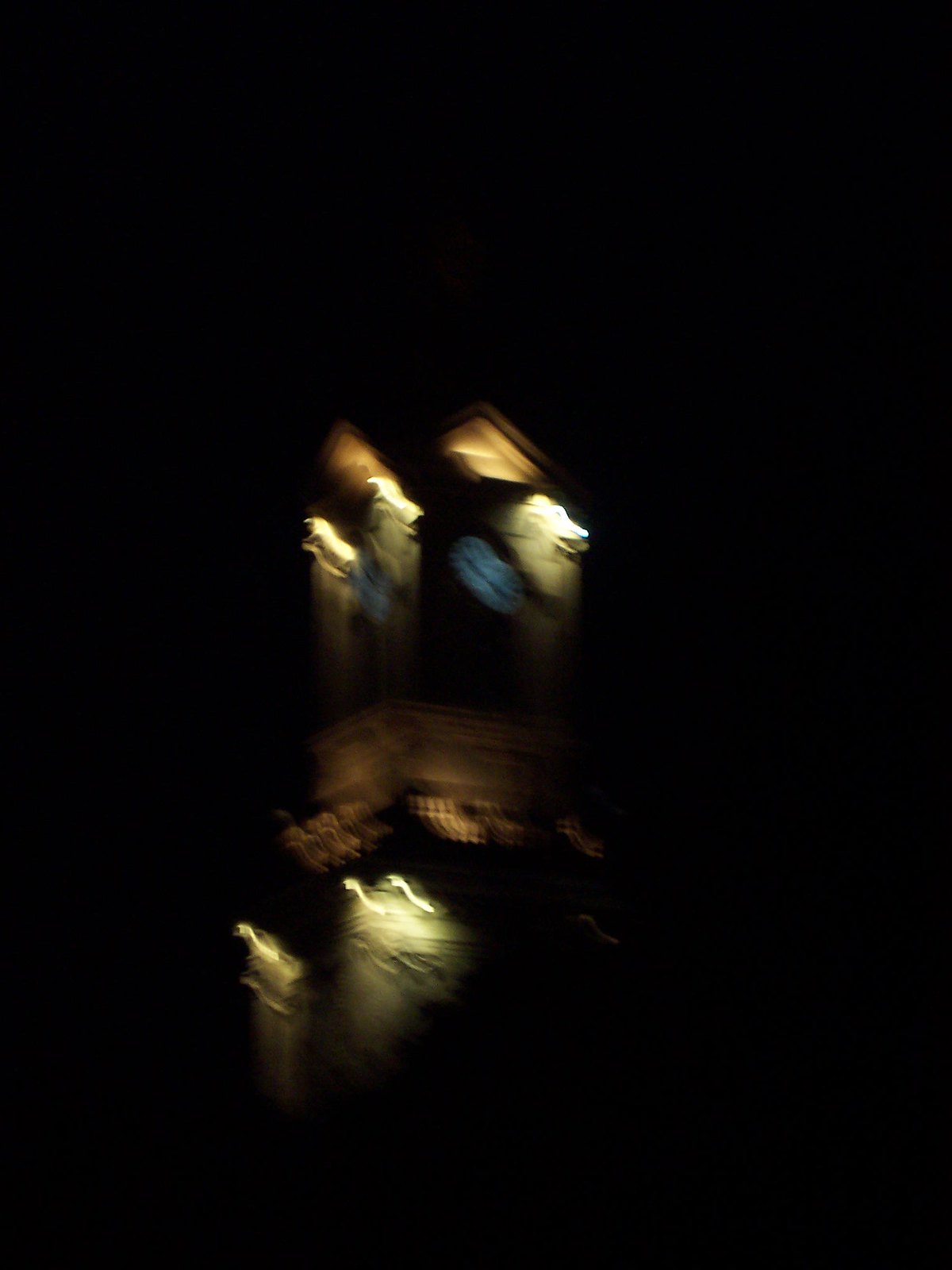A nighttime photograph captures a blurry image of a tall, steeple-like tower, part of a larger unseen building. This tower, set against an otherwise pitch-black background, features sporadic lights that appear to illuminate various architectural elements, possibly gargoyles or other ornate decorations. The image is dominated by white and yellowish lighting that highlights parts of the structure, mixed with patches of blue light, giving an impression of either abstract forms or animal-like faces. Despite its subdued colors—whites, grays, and browns—the stone-like textures and the lights create an eerie, mysterious presence. A distinct blue phenomenon resembling a microorganism can be seen on the lens, adding to the otherworldly feel. The overall blurriness suggests the photograph was taken with a moving camera, enhancing the ghostly atmosphere of the scene.